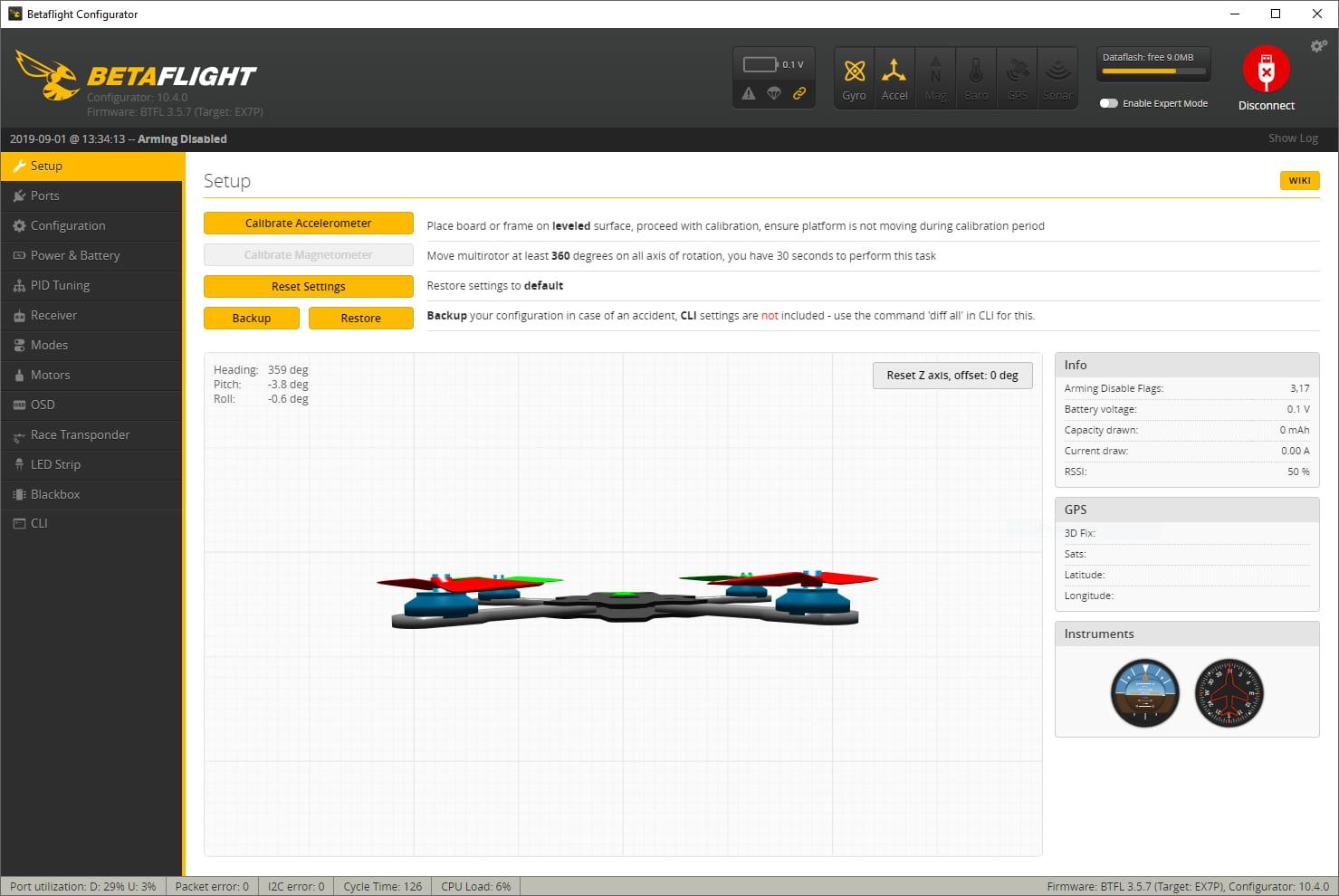The image at the top features a yellow graphic resembling a helicopter or wing, accompanied by the text "BetaFlight" — where "Beta" is in yellow and "Flight" is in white. Below this, there's a section labeled "Setup" and options for "Reset Settings," "Backup," and "Restore," all highlighted in yellow rectangles. Below, there is an image of a streamlined drone or remote-controlled flying device with four extensions stemming from the center, each topped with blue oval shapes and propellers. The front two propellers are red, while the rear ones are bright green. To the right, there are labels "Info" and "GPS" set against a gray rectangle background, along with "Reset Z Axis Offset" also within a gray rectangle. In the upper right corner, there's a red circle featuring an icon of a USB plug with an X in the center.